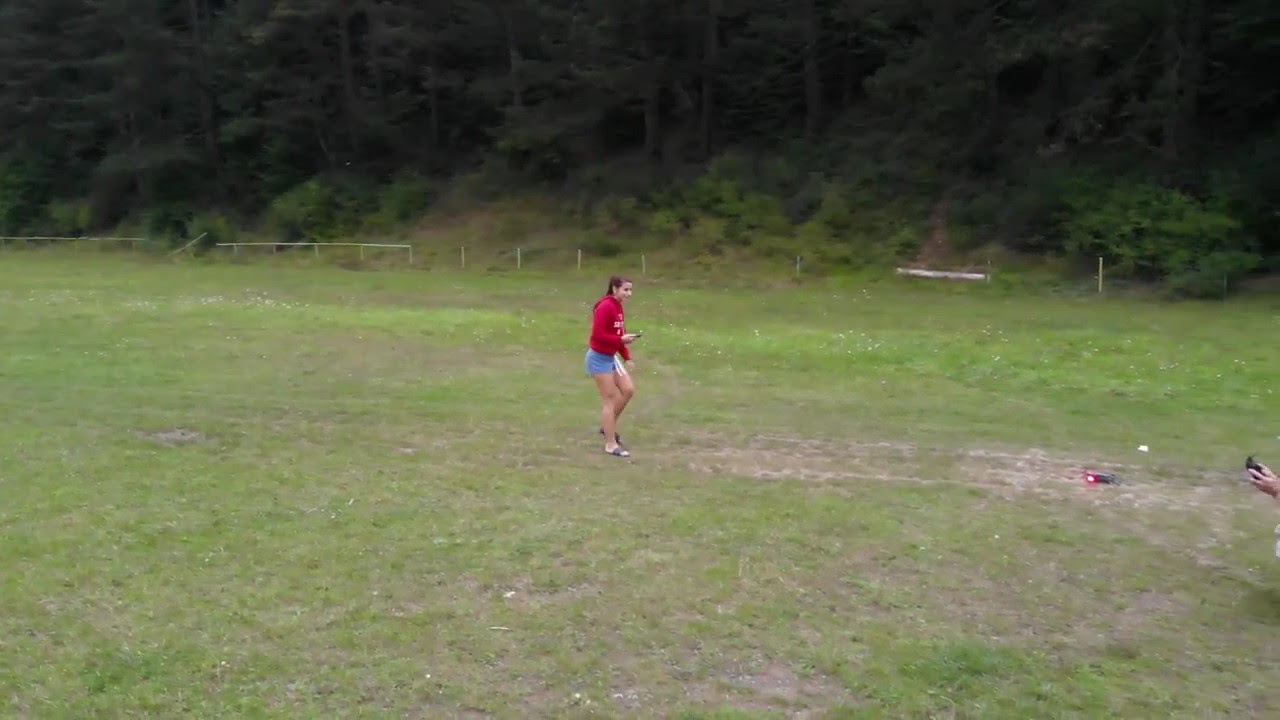In this photo, on an overcast summer day, a young teenage girl, around 16 or 17 years old, is captured in motion in the center of a muddy, grassy field with sporadic dirt patches. She has brown hair tied back in a ponytail and is wearing a red hooded sweatshirt with long sleeves, paired with blue shorts and brown flip-flops. She is holding a cell phone in her right hand and appears to be stepping through the mud. Approximately 15 feet in front of her on the ground, there is a small black device with a red illuminated light. The background reveals a dilapidated white fence, partially intact on the left side but broken on the right, likely overtaken by natural elements over time. Behind the fence, dense green shrubs and trees suggest the edge of a forest. On the far-right edge of the image, a hand partially visible appears to be holding a camera, possibly taking a picture of the girl.